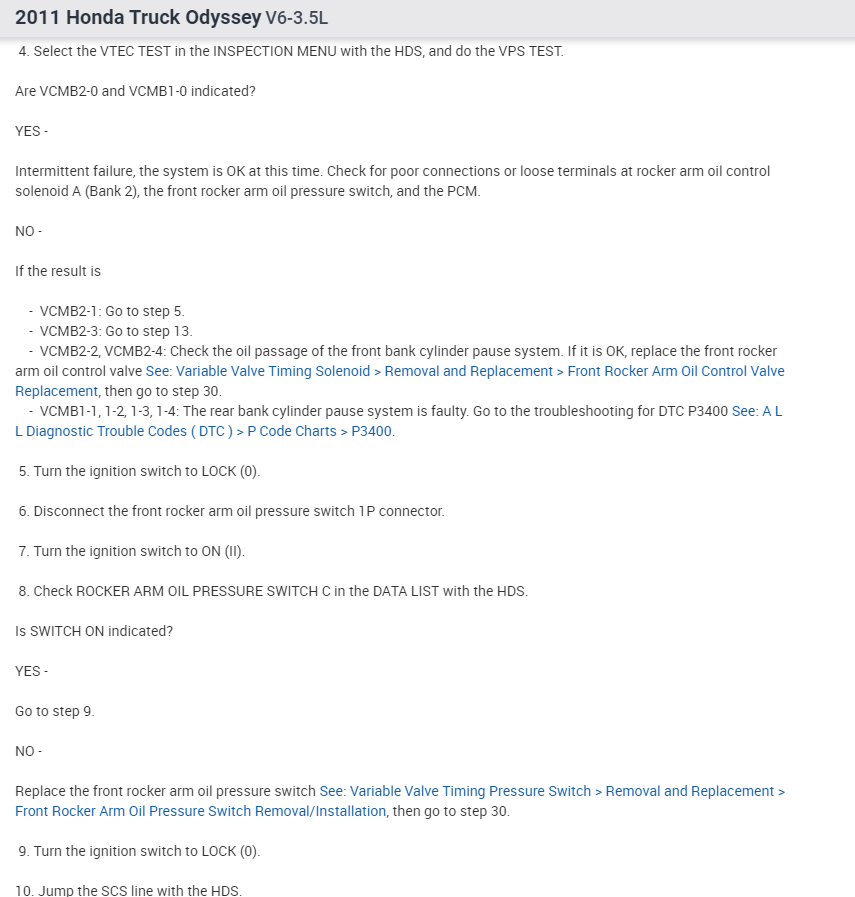### Detailed Caption:

This image displays a screenshot from an article or web page providing detailed instructions on troubleshooting and resolving issues with the variable valve timing and lift electronic control (VTEC) system of a 2011 Honda Odyssey Truck with a V6 3.5L engine. At the top of the screenshot, there is a grey bar containing the text "2011 Honda Truck Odyssey V6 3.5L VTEC." Below this, a white background is filled with step-by-step instructions. 

The instructions primarily focus on using the Honda Diagnostic System (HDS) to perform various tests and checks. The specific steps include:
1. Selecting the VTEC test in the inspection menu on the HDS and performing the VPS test.
2. Analyzing the results to determine if VCM V2.0 or VCM V1.0 are indicated.
   - If "Yes," it signifies an intermittent failure, and the system is currently functional. Further instructions include checking connections or terminals at specific components such as the rocker arm oil control solenoid A (Bank 2), the front rocker arm oil pressure switch, and the Powertrain Control Module (PCM).
   - If "No," alternative steps (5, 13, or 30) are outlined depending on the VCBM (Variable Cylinder Management) codes received (e.g., VCBM 2.1, 2.3, 2.4).

Additional steps detail specific actions, including turning the ignition switch to various positions, disconnecting connectors, checking switches, and replacing faulty components like the front rocker arm oil control valve or pressure switches. Detailed diagnostic procedures and troubleshooting for different VTEC related codes (e.g., DTCP3400) are also provided.

This comprehensive guide is a concise yet detailed resource for diagnosing and addressing VTEC system issues in the specified Honda vehicle model.